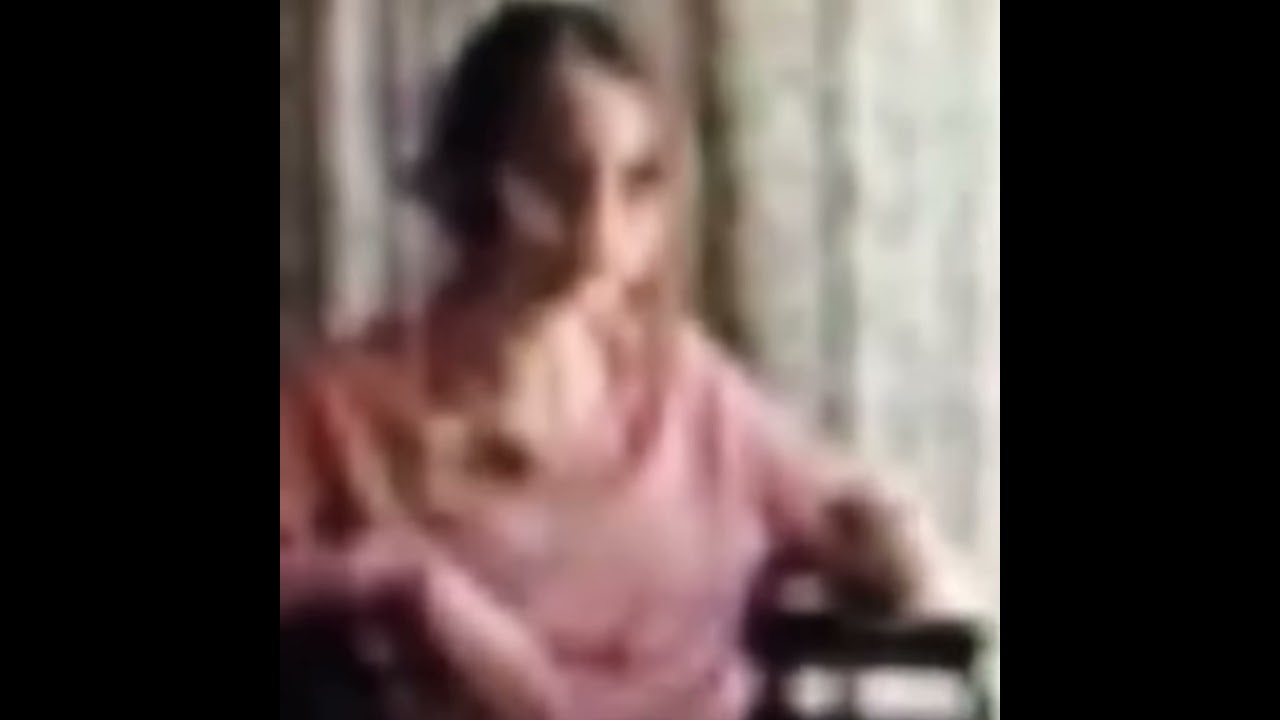The image is extremely blurry, making it difficult to discern details clearly. In the center, there appears to be a woman, either elderly or young, with medium-length black hair that might be tied in a ponytail. She is wearing a pink sweater and is seated in a black chair, identifiable from the partial view of the black hand rests where her elbows rest. The woman is positioned slightly towards the left but mostly centralized, and her facial features are indistinct. The background is uniformly white with no discernible objects, and there are solid black borders on both the left and right sides of the image. Strong white lighting seems to be coming from the upper right. The overall quality of the image is poor, making it hard to determine the exact setting, but it evokes a sense of melancholy as the woman appears to be looking off to the side, not directly at the camera.